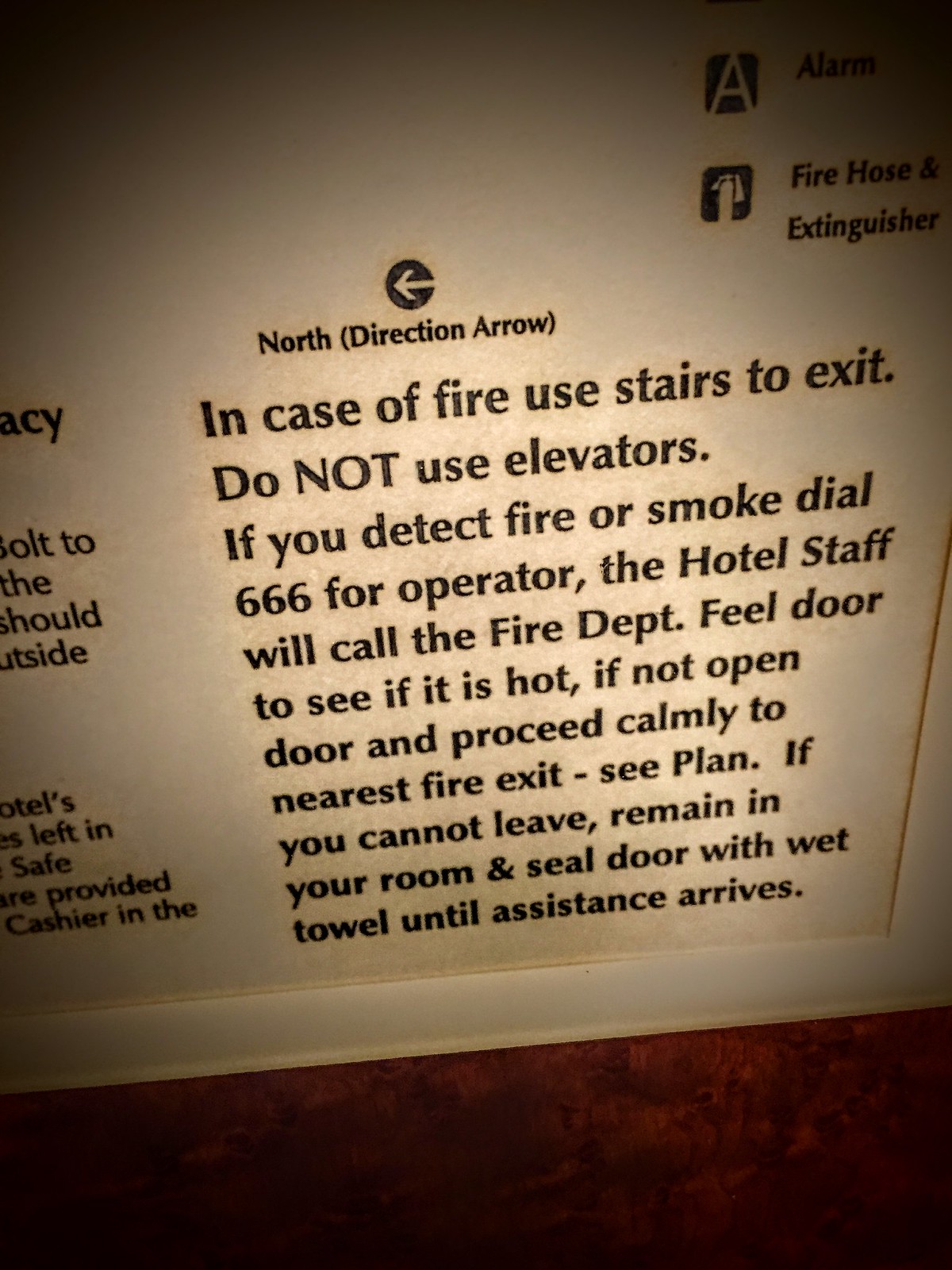The image depicts an informational fire safety sign posted on the wall at what appears to be the ground-level area of a hotel, indicated by a white border separating the wall from the floor. The sign, centrally positioned and clearly visible, features a detailed set of instructions in black text against a white background. At the top left, there is a black circle encasing a white arrow pointing left, labeled as "North (Direction Arrow)." To the right, two icons are present: one representing an alarm and the other a fire extinguisher labeled "Fire Hose and Extinguisher."

The instructions read: "In case of fire, use stairs to exit. Do not use elevators. If you detect fire or smoke, dial 666 for operator. The hotel staff will call the fire department. Feel door to see if it is hot. If not, open the door and proceed calmly to the nearest fire exit. See plan. If you cannot leave, remain in your room and seal door with a wet towel until assistance arrives." The sign is designed to provide clear and concise safety information to hotel guests, ensuring they know the procedures to follow in the event of a fire. The colors featured in the sign include red, white, black, tan, and yellow, adding to its visibility and urgency.